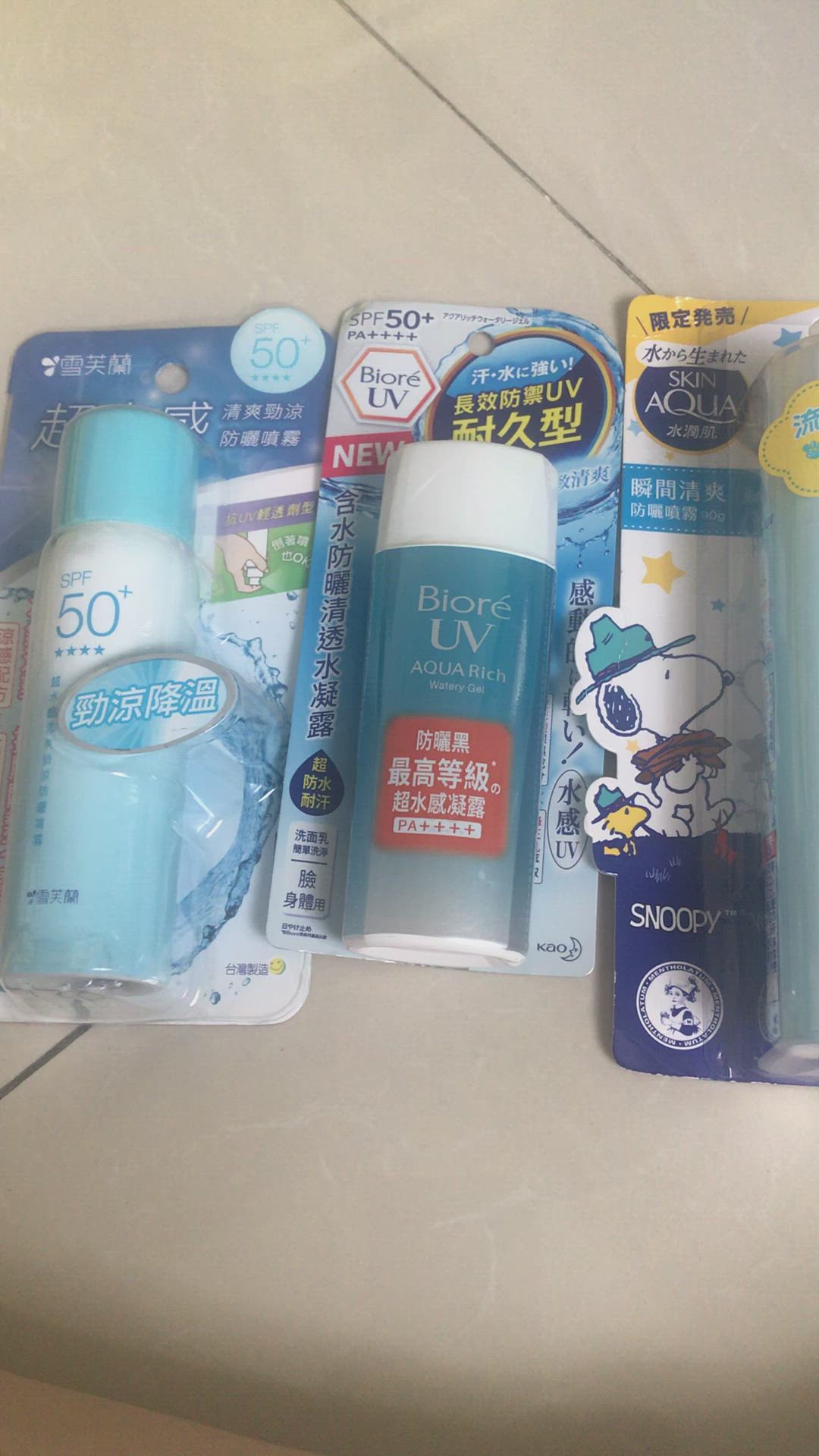A display of suntan and sunblocking lotions in bubble pack and cardboard packaging, designed for hanging on a rack in a store. The primary language on the packaging is Chinese, with some English text. 

- On the left, a light blue, spray bottle prominently displays "SPF 50+" along with various Chinese text. The cardboard backing includes an illustration showing the bottle being held upside down while spraying. 
- The middle product is labeled "Bio-Ray UV Aqua Rich..." in English, with additional Chinese inscriptions covering the majority of the information. The bottle appears to be white, encased in a bluish-gray shrink-wrap label, and topped with a white cap.
- Although mostly off-frame, the third product's packaging shows a "Skin Aqua" label and an image of Snoopy, the iconic dog, carrying firewood and wearing a ranger hat, accompanied by his bird friend in matching attire. The "Snoopy" trademark is also visible, and the edge of a light blue bottle can be seen beneath the plastic packaging.